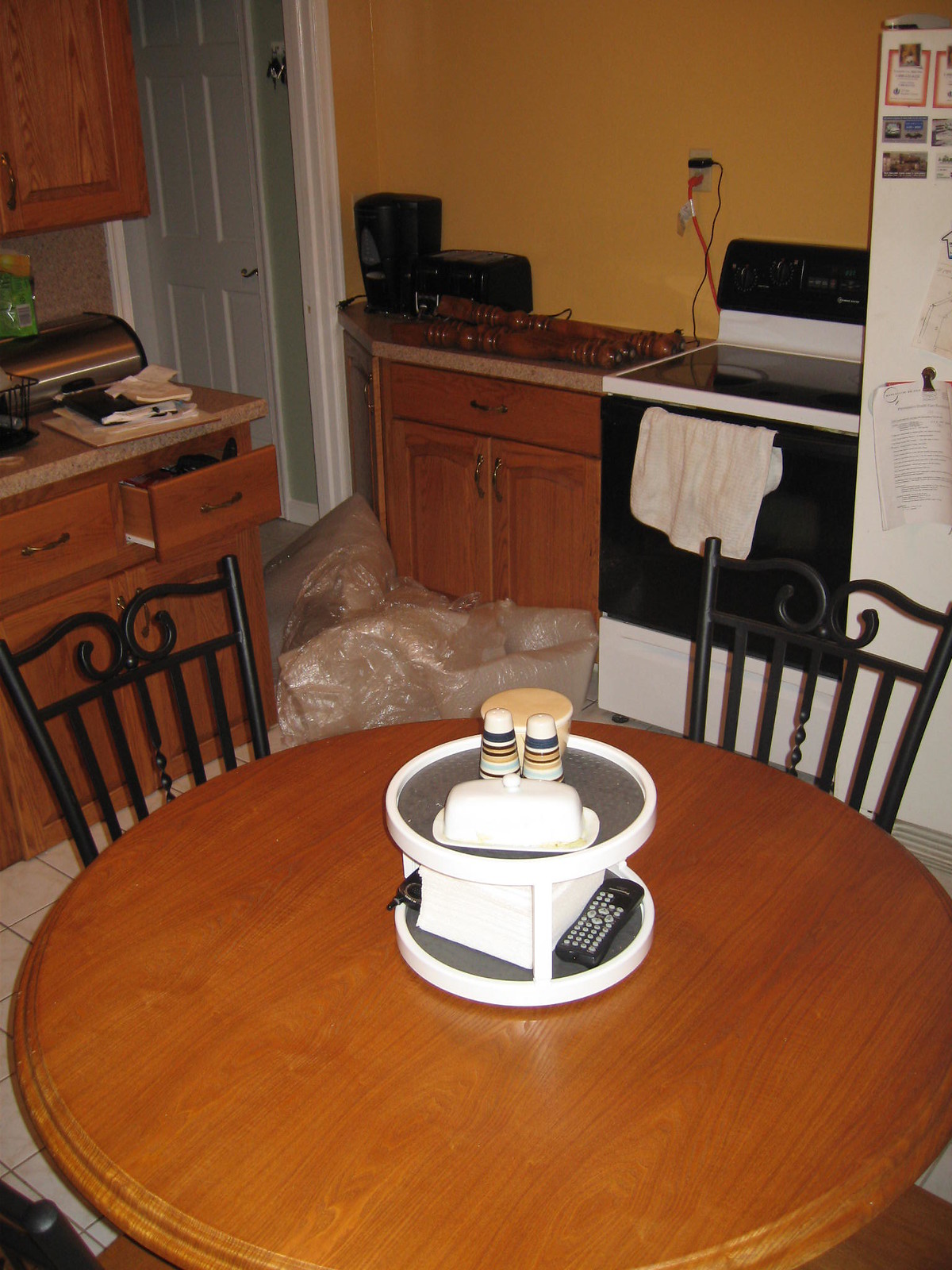This photograph showcases a kitchen interior that evokes the classic aesthetic of the late 1970s to early 1990s. The cabinets are a defining feature, with their period-specific design and coloration that complements the overall retro ambiance. The kitchen includes era-appropriate appliances, prominently featuring a white electric stove with a smooth cooktop and dark trim, along with a unique dark oven door adorned with a white towel hanging from the handle. The adjacent white refrigerator continues the vintage theme.

On the countertop to the left of the stove, various small appliances are visible, potentially including a vintage radio and a coffee maker, alongside what appears to be wooden spindles from furniture. A round table occupies the center of the room, encircled by new wrought iron-style chairs, whose design suggests affordability.

Atop the table sits a white double-decker Lazy Susan, with a TV remote control stored on the lower tier. The assortment on the table also includes a small two-way radio antenna peeking from behind a stack of napkins, hinting at a setting where maintaining communication is essential, possibly a farm. Other items on the table include a butter dish and salt and pepper shakers.

The kitchen's countertops feature additional details such as a bread storage box and scattered papers, enhancing the lived-in feel. The floor is covered in older tile, reinforcing the kitchen’s vintage charm. In the background, a white door leads to a hallway, providing an exit from this nostalgic culinary space.